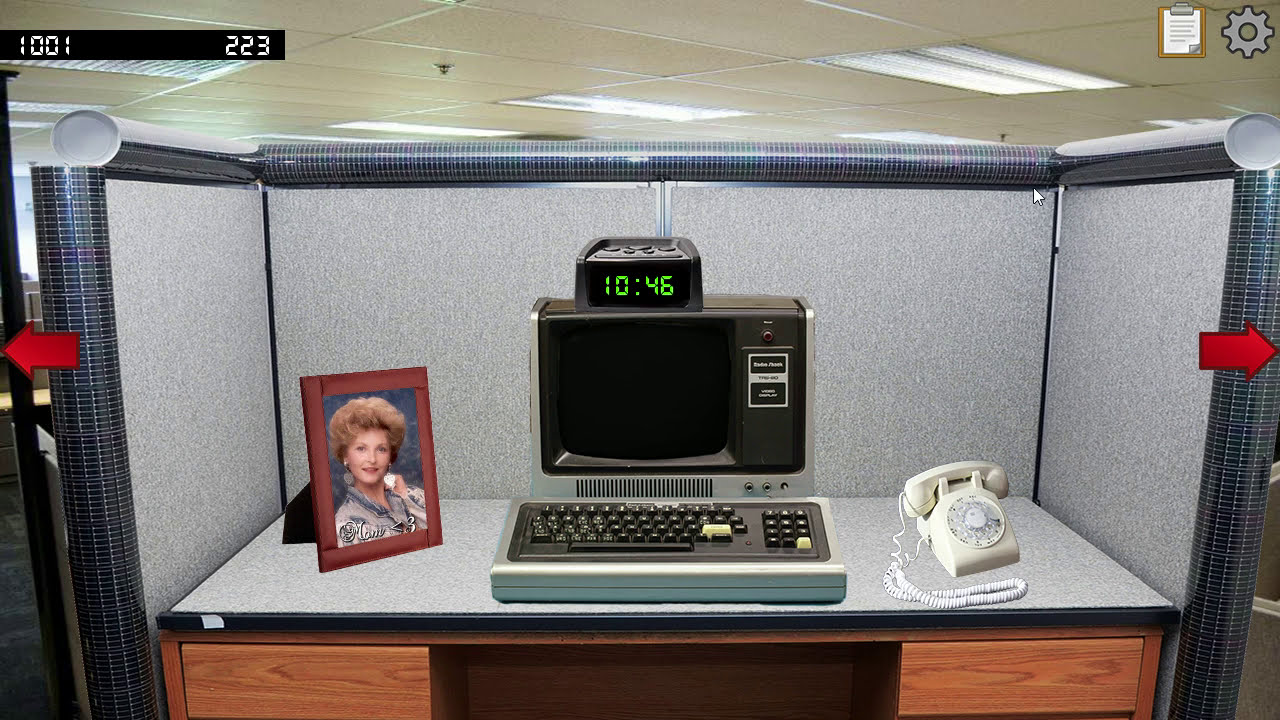This horizontal rectangular image depicts a screenshot from a video game, characterized by numerical indicators "1001" and "223" at the top center against a small black rectangular background. Additional game icons, a clipboard, and a settings button occupy the upper right corner. Central to the scene is an elderly office cubicle with gray walls and a low ceiling illuminated by fluorescent lights. Dominating the scene is an old-fashioned computer, reminiscent of technology from the late 1970s to early 1980s, featuring a boxy CRT monitor with black and silver detailing, accompanied by a thick keyboard. Situated atop the monitor is a sizable digital alarm clock displaying "1046" in green digits. To the left of the computer rests a picture frame with a photograph of a woman, while to the right sits a white rotary dial telephone with its trademark cord. The desk itself, a wooden surface with brown drawers, supports this retro equipment. On either side of the screen, red arrows point left and right, enhancing the electronic display's interactive nature.